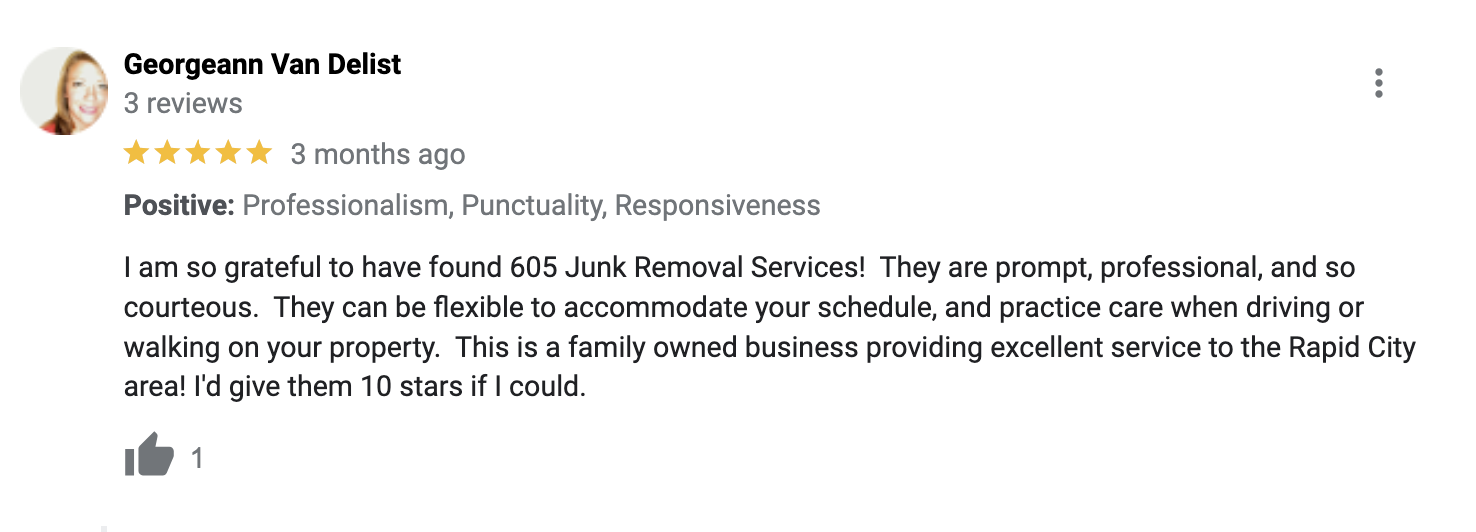On a white background, there is an image of a white female with dirty blonde hair encased in a grey circle. Positioned in black font above her image are the names "George and Van de List." Below this, "Three Reviews" is written in grey font, followed by a display of five yellow stars. Continuing down, "Three Months Ago" appears in grey font with the words "Positive, Professionalism, Punctuality, Responsiveness" underneath.

The text of the review reads: "I am so grateful to have found 605 Junk Removal Services. They are prompt, professional, and so courteous. They can be flexible to accommodate your schedule and practice care when driving or walking on your property. This is a family-owned business providing excellent service to the Rapid City area! I'd give them 10 stars if I could."

Additionally, there is a grey hand with a grey cuff giving a thumbs up, beside which is the number 1 in grey. On the far right of the name is a vertical line of three white dots.